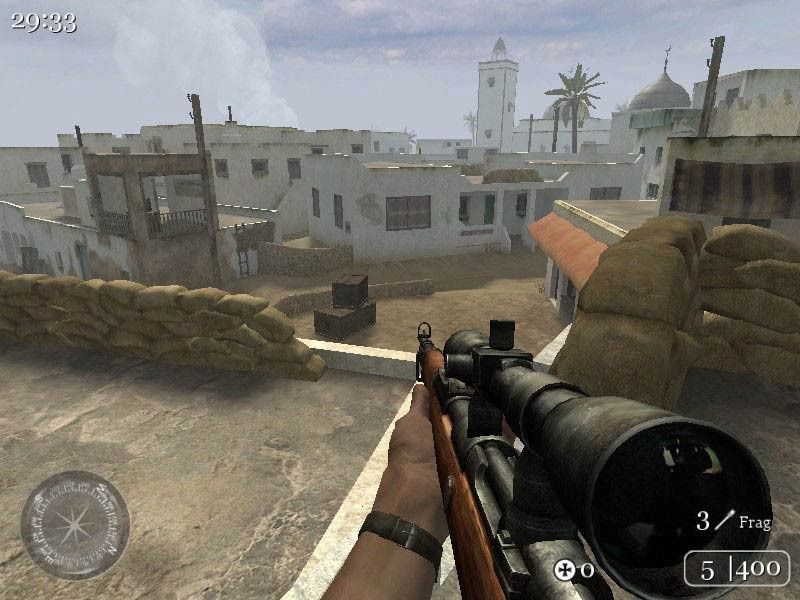The image appears to be a screenshot from a first-person shooter video game. In the upper left corner, there is a timer showing 29 minutes and 33 seconds. The scene is viewed from the perspective of a player holding a sniper rifle, overlooking a cityscape that evokes a Middle Eastern setting. All the buildings are white with some palm trees interspersed. The ground features a mix of stone-like surfaces and sandbags neatly stacked up. The vantage point suggests the player is standing on a flat rooftop, peering down at several crates below. Although no characters are visible in this frame, there seems to be a small area with railings resembling a watchtower, possibly harboring someone. The sky is overcast. The sniper rifle's display at the bottom of the screen shows ammunition details, indicating five rounds, a range of 400 meters, three additional items, and a grenade symbol labeled "frag". In the bottom left corner, a compass is also visible, aiding navigation.